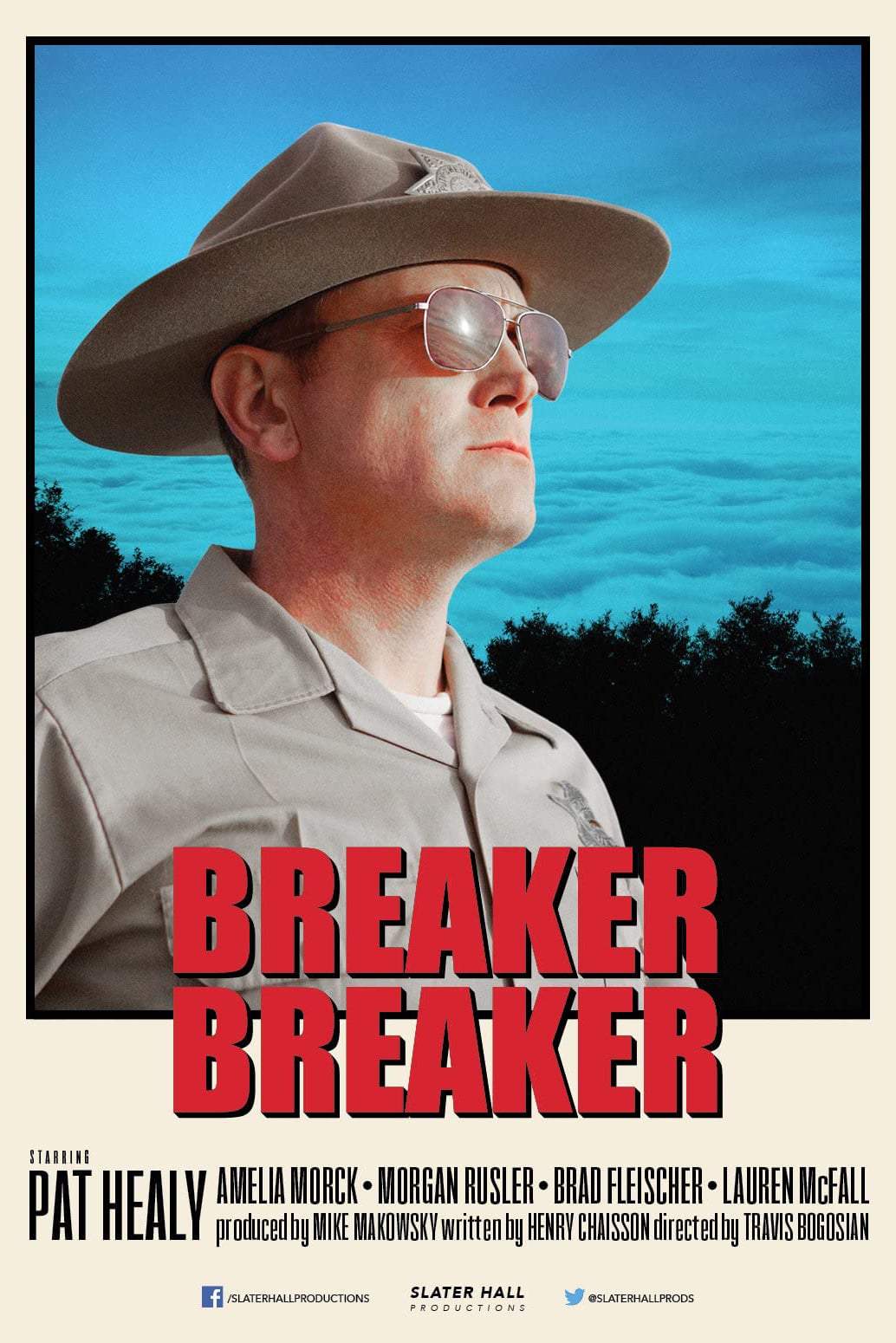The movie poster for "Breaker Breaker" prominently features a rugged white man in profile, who appears to be a forest ranger or law enforcement officer. He dons a Smokey the Bear-style ranger hat with a wide brim and aviator sunglasses, exuding a stoic demeanor as he gazes slightly away from the camera. His outfit includes a khaki button-down shirt layered over a white t-shirt, complemented by what seems to be a badge or emblem on his left breast. The setting behind him is an outdoor forest scene during the daytime, with silhouettes of trees against a backdrop of white clouds and a dark blue sky.

At the top of the poster, the bold red text reads "Breaker Breaker." Below that, in descending order, the black text lists the cast and crew: "Starring Pat Healy, Emilia Mork, Morgan Rusler, Brad Fleischer, and Lauren McFaul. Produced by Mike Mikowski, written by Henry Chaisson, and directed by Travis Boghossian." The production company, Slater Hall Productions, features prominently alongside social media icons, with the Facebook logo and Slater Hall Productions text on the left, and the Twitter bird icon with the handle @SlaterHallProds on the right.